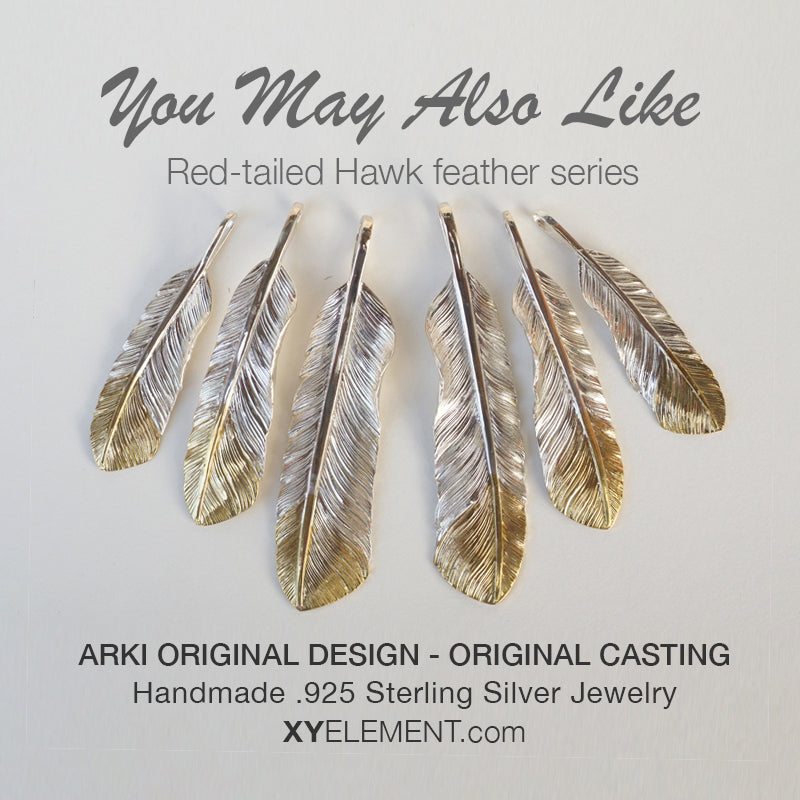This advertisement from xyelements.com presents the ARCHE original design "Red-Tailed Hawk Feather Series," featuring beautifully crafted 0.925 sterling silver feathers. The display showcases six feathers, arranged in a visually appealing manner, with two large feathers in the center, flanked by progressively smaller ones. Each feather is meticulously handcrafted, with the main body in silver and the tips elegantly dipped in gold. The sophisticated advertisement is set against a plain grey background and includes a headline in bold cursive writing, "You May Also Like," highlighting the exquisite and timeless design of these handmade treasures.